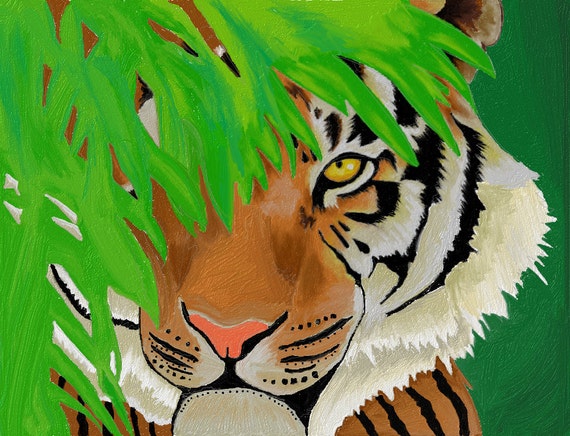The image is a small, four-inch wide by three-inch high painting of a tiger on canvas. The composition features an abundance of green branches and leaves from a tree, which extend from the upper left corner to the lower left corner and continue almost to the right edge before flowing downward at a leftward angle. These green elements partially obscure the tiger's face, covering its left eye and ear. Visible in the upper right corner is the right ear, while the yellow right eye is surrounded by black, transitioning into the white cheek area marked with black stripes. The tiger's nose and muzzle are a striking orange, with a notably pink nose and black whiskers. The background on the right side of the image is painted in a dark green hue, complemented by a touch of tan color above the tiger's head. The tiger appears to be simply gazing outward, with no indication of aggression or movement.